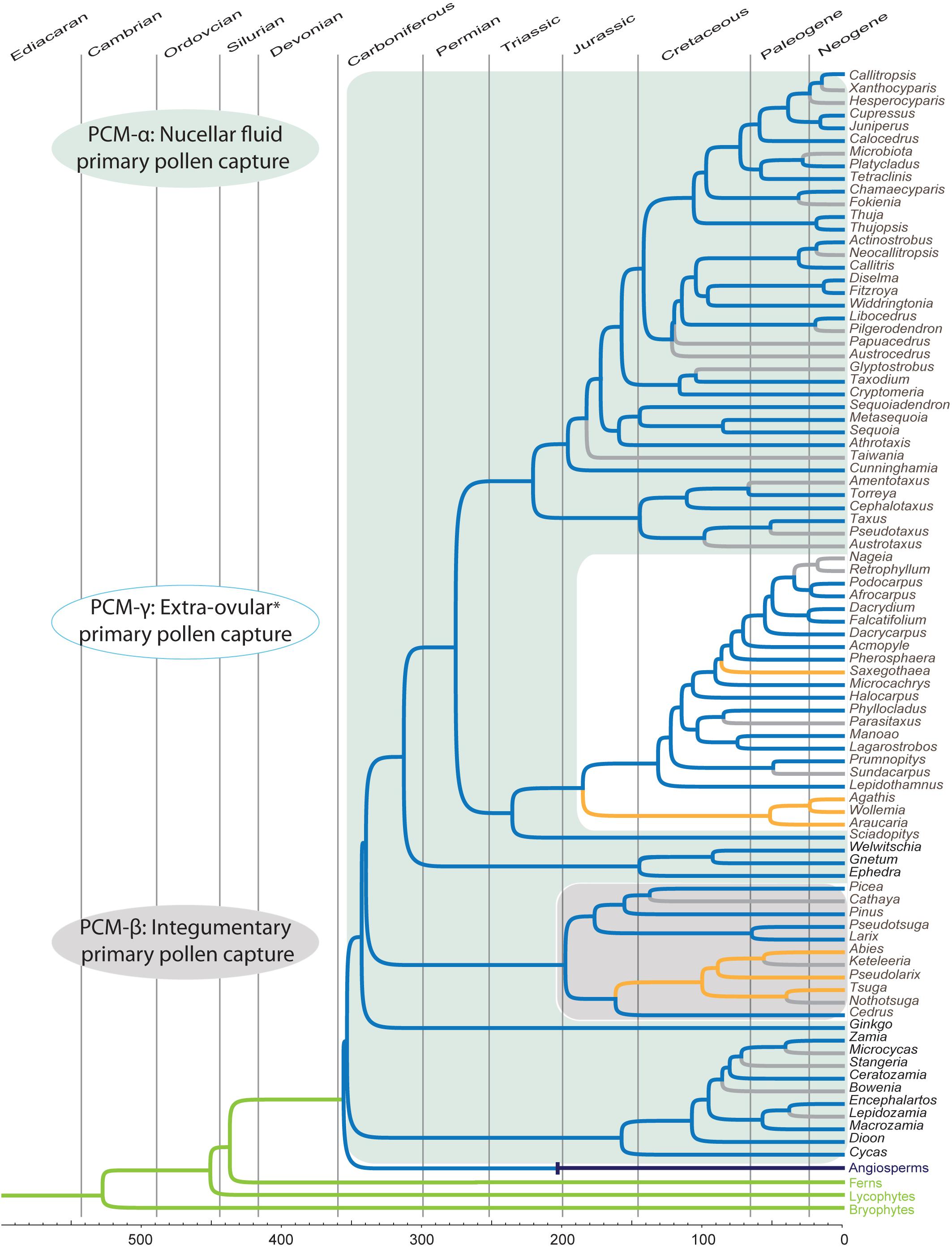The image depicts a complex, computer-generated biological chart with a light mint green background. It is organized into three primary categories: PCM-A, PCM-Y, and PCM-B, representing different types of primary pollen capture systems—new cellar fluid primary pollen capture, extra ovular primary pollen capture, and intergemunitary primary pollen capture, respectively. Dark teal lines extend down the image, connecting numerous text labels. The chart's vertical layout features ellipses corresponding to PCM Sigma at the top, PCM Gamma in the center, and PCM Beta at the bottom. Additionally, each category is linked to specific text labels on the right side through a network of lines in varying colors, including blue, yellow, and gray. Across the top, there are labels for different geological eras or eons such as Kidakere, Cambrian, Ordovician, Silurian, and Devonian. At the bottom of the chart, a scale measures time frames in years, marked from 500 to 0, illustrating the temporal distribution of pollen types and their capture mechanisms.